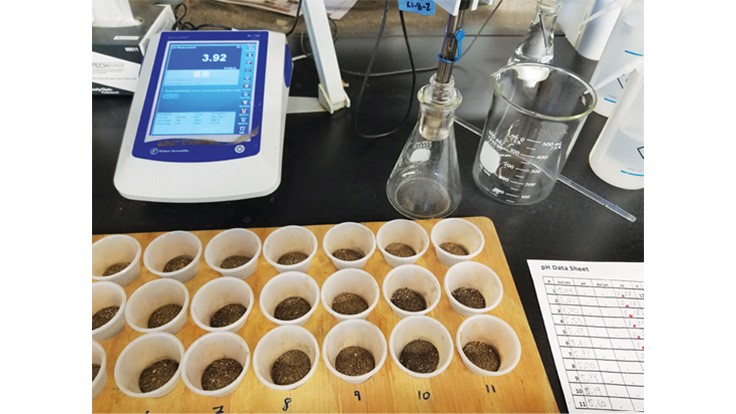In this image, a black table serves as the workspace. On the bottom left, there is a brown board arranged with clear cups in rows, each row containing seven cups for a total of 21 cups. These cups appear to hold small brown bits. The cups are labeled with numbers, progressing from left to right in the back row starting with 11, 10, 9, 8, 7, 6, 5, and the numbering continues off-image.

Positioned above the brown board, there is a white device featuring a prominent blue screen. The screen displays the number "3.92" in white font against a deeper blue background, accompanied by additional blue imagery to the right and a lighter blue section just below.

To the right of this device, there are clear glass flasks. One of these flasks contains metal tubing, while the second flask stands alone. Adjacent to these, there is a clear glass mixer. More clear bottles are situated at the top right side, each marked with blue lines above and underneath.

In the background, black cords are visible, adding to the laboratory setup. Also present is a white sheet of paper with black lines, titled "pH Data Sheet," suggesting it contains relevant data for the experiments shown on the table.